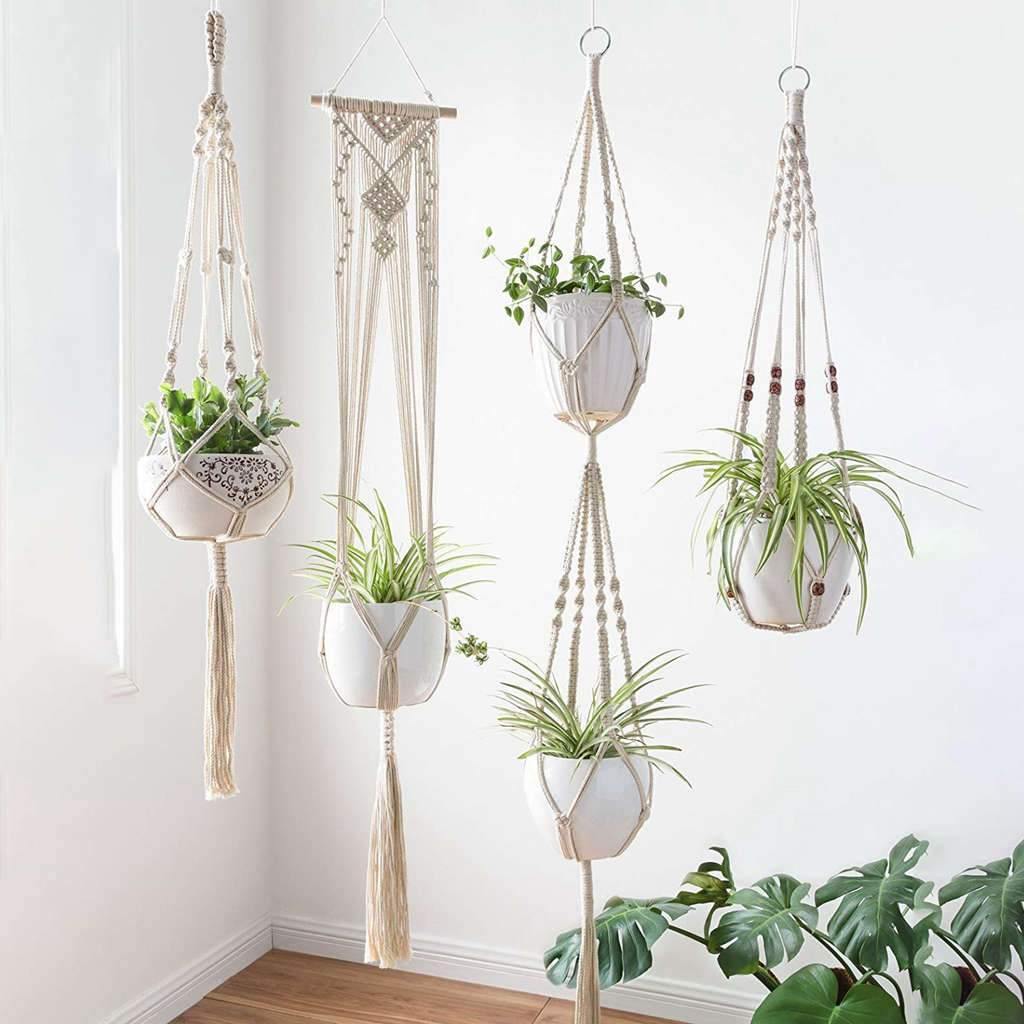This image depicts a vibrant, sunlit room with solid white walls and medium-colored hardwood floors. The photo captures a cozy corner of the room where four white planters, each hanging from the ceiling with intricate white macrame holders, are prominently displayed. The macrame holders exhibit a bohemian woven weave design, which securely cradles the planters. The planters contain lush greenery, including spider plants and ivy-like vines, with tassels hanging from three of them, adding to the decorative appeal. To the bottom right of the image, a large leafy green plant in a container partially enters the frame from the floor, contributing to the room's fresh, serene ambiance.